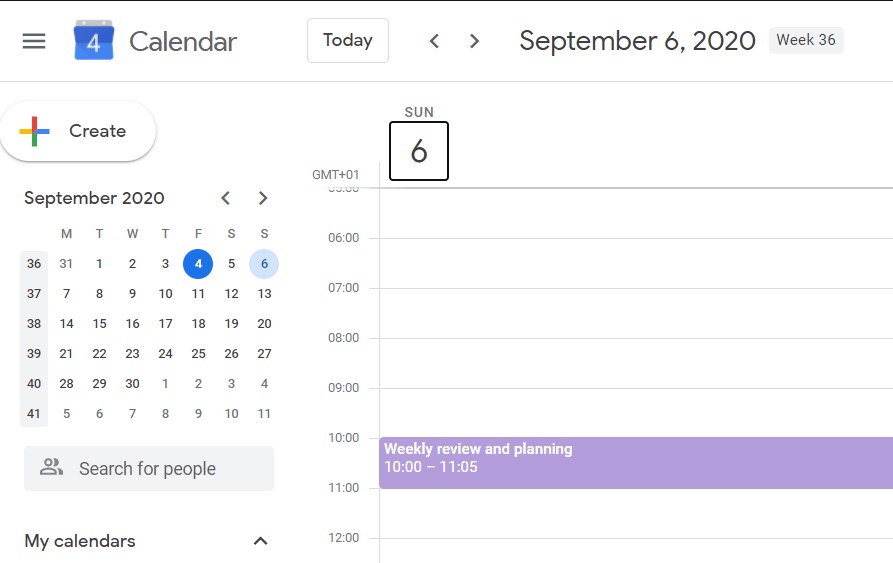This is a detailed screenshot of a Google Calendar layout. At the very top of the image, there is a stark white background with a black vertical line intersecting a black horizontal line. Beneath these lines, a blue calendar icon with the number "4" prominently displayed is accompanied by the word "calendar" in black font. Moving to the right, there is a black-outlined rectangle containing the word "today" in black font, flanked by small arrows that allow the user to navigate between days.

The main date displayed is "September 6th, 2020," and it is noted as "week 36" of the year. On the left side of the image, a mini-calendar shows the entire month of September 2020 with days organized from Monday to Sunday. Below this mini-calendar, there are options to "search for people" and access "my calendars."

The right section of the calendar is dedicated to event details. It displays "Sunday the 6th" along with the time zone "GMT +01." The calendar is depicted from 6 AM to 12 PM, with a specific event, "Weekly Review and Planning," scheduled between 10 AM and 11 AM.